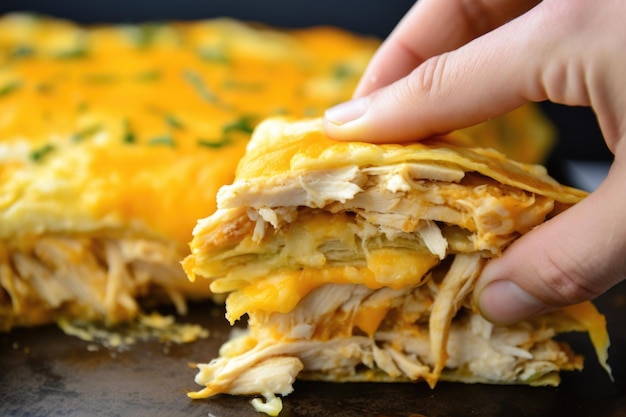The image showcases a vibrant, multi-layered quesadilla, prominently featuring layers of succulent white meat, likely chicken, and melted cheese, all encased within golden tortillas. The quesadilla is presented on a black surface, with most of it visible in the background, slightly blurred to draw attention to the foreground slice. This slice reveals the intricate layering: starting with a base tortilla, topped with alternating layers of tender chicken breast, gooey cheese, and more tortillas. A hand is shown pressing down on the top tortilla, allowing a clear view of the rich, melty cheese, and slices of chicken breast, accented by green chives. The combination of textures and colors, from the creamy white meat to the vibrant yellow sauce interspersed within, creates a mouth-watering display of this traditional Mexican dish.